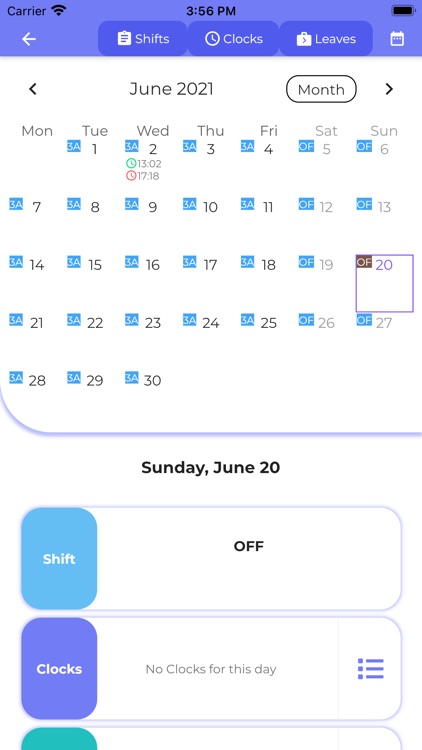Here is a refined and detailed caption for the image based on the provided description:

---

The image is a screenshot from a smartphone displaying a scheduling application. The top of the screen features a rectangular label in a light blue to lavender hue, with the top left corner displaying the word "carrier" alongside full Wi-Fi signal bars. The time reads 3:56 p.m., and there is a back arrow button in the top left corner.

Directly below, there are three darker blue rectangular buttons labeled "Shifts," "Clocks," and "Leaves." Beneath these buttons is a calendar layout for June 2021, with individual boxes representing each date. Specifically, on June 2nd, there are two entries: one marked in lime green and the other in red. On June 20th, a purple box indicates the date with the label "Off."

Below the calendar, daily details for Sunday, June 20th are displayed. This section includes circular rectangular buttons: "Shifts" in blue, "Clocks" in a lavender shade, and a partially visible teal button at the bottom. The "Shifts" button is labeled "Off," and the "Clocks" button has a note saying "No clocks for the day." There is also a three-line menu option for additional settings. The calendar section dominates the top portion of the screen.

---